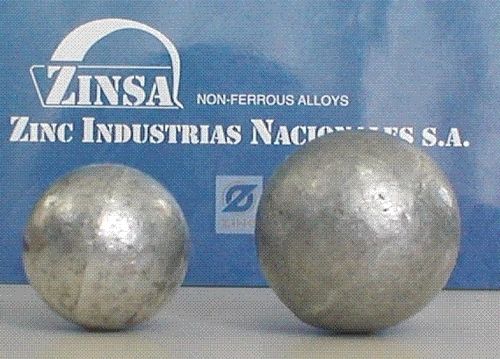The image displays two smooth, silver zinc balls positioned side by side on a gray surface. The ball on the right is larger than the one on the left. Both balls, which have a somewhat dull but reflective finish with patches of light due to illumination, resemble bowling balls without any holes. Behind the balls is a blue panel featuring white text and a logo. The text reads "Zinsa" with a swooping swirl-like design above it, followed by "Non-Ferrous Alloys," "Zinc Industrious," and partially hidden text starting with "N" and ending with "SA" due to the larger ball's position. Between the balls on the wall, there is a white square containing a blue circular logo with a diagonal line through it.